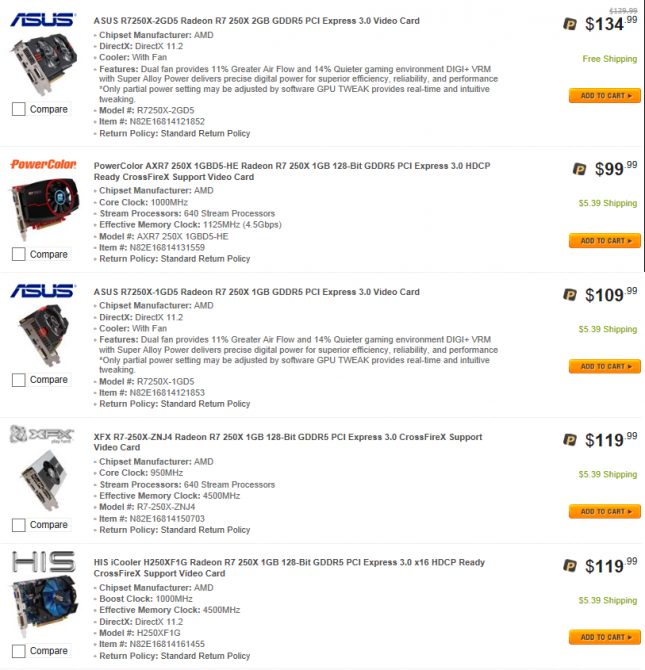The web page displays a selection of video cards available for purchase, laid out in a structured and detailed manner. On the left-hand side, there are images of five different video cards. Adjacent to the images, detailed descriptions of each video card are provided, listing their specifications and features. Further to the right, the prices are displayed for easier comparison. 

The first option is an Asus 3.0 video card, interfaced through PCI Express, priced at $134. Directly below it is the PowerColor AXR7, available for $99. The third choice is another Asus model, the Radeon R7, equipped with 1 GB of memory, making it a more affordable option at $109. The fourth option is an XFX R7, featuring Crossfire X support, priced at $119. Finally, the bottom option is the HIS iCooler Radeon R7 video card, noted for being MDCP ready, also priced at $119. Each video card listing includes a square checkbox, allowing buyers to select and compare multiple cards directly on the page.